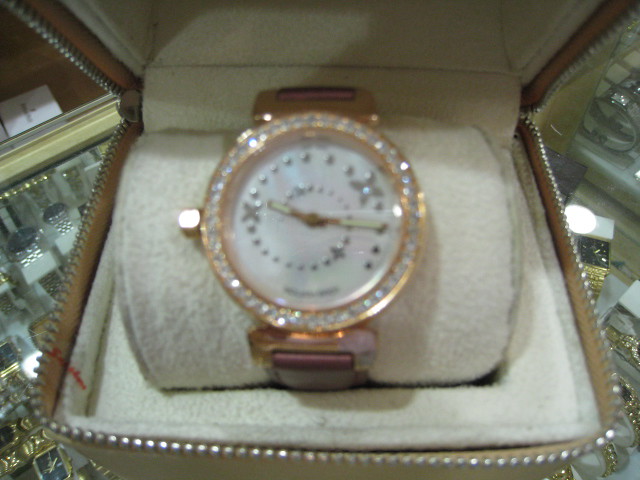This color photograph features a luxurious watch displayed in a high-end jewelry box. The box itself is adorned with diamonds or possibly cubic zirconias, adding an air of opulence. The interior of the box is lined with a tan or cream-colored fabric, designed to enhance the watch's elegance. The watch, with a golden exterior, is encrusted with sparkly crystals around the bezel and within the dial, which features intricate patterns that resemble butterflies or Chinese star weapons. It is 9:15 on the watch, with luminous, golden minute and hour hands. The watch face is white, surrounded by a spiral design and accented with dotted silver lines indicating the hours. The watch is fastened with maroon leather straps and includes a golden knob on the side. Positioned on top of a glass display case in the photograph, the watch is framed by a collection of other timepieces inside the case below. You can see the reflection of a light in the glass, highlighting various silver and gold watches neatly arranged within, creating a sense of refinement and luxury.